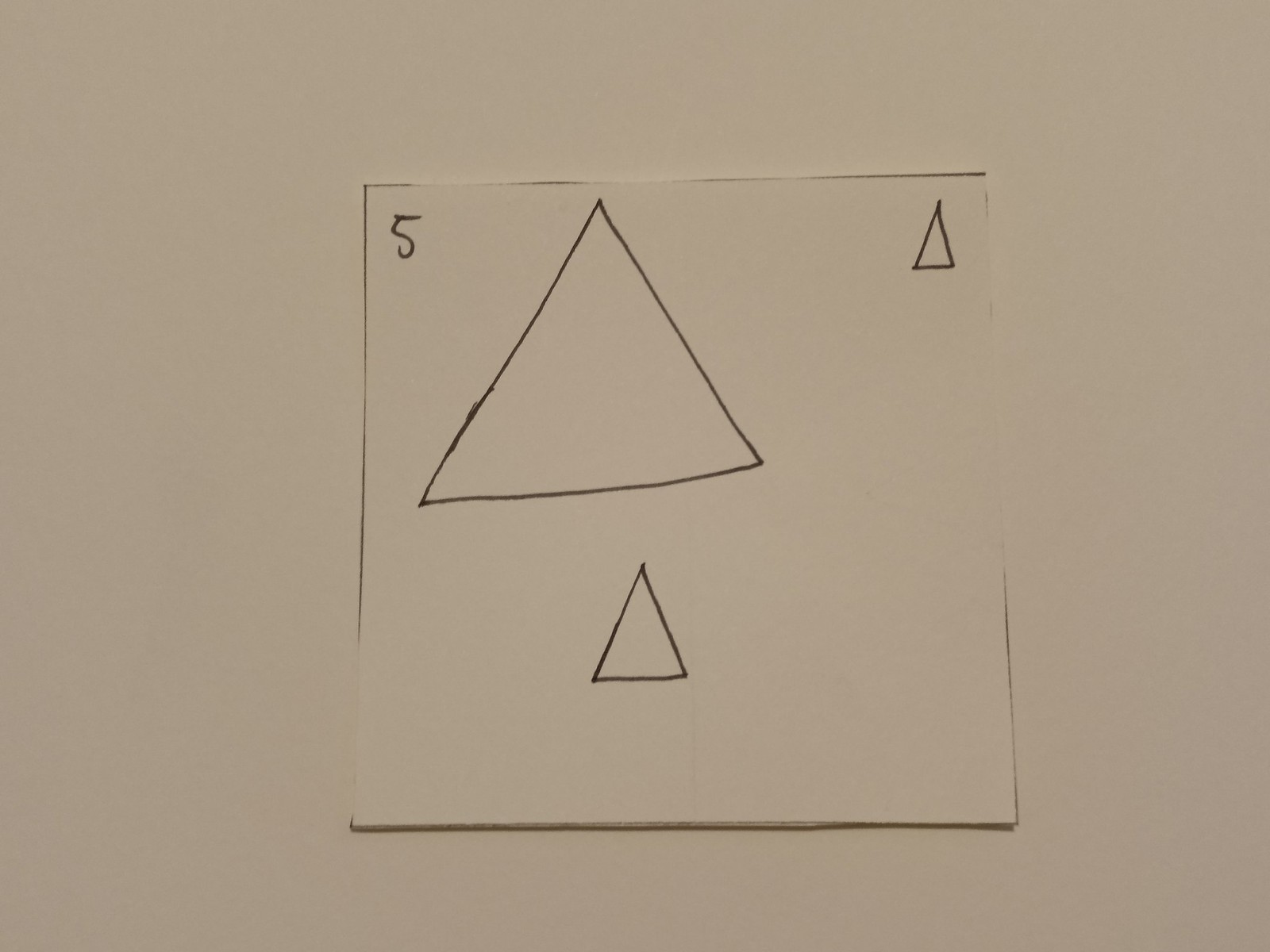The photograph features a square piece of white paper or thin card set against a pristine white background, which could be a wall, floor, or another sheet of paper. The square piece has visible guide lines indicating where it was cut, with some remnants of these lines still present, revealing that the trimming was not entirely precise. A subtle shadow along the bottom edge of the square suggests that the material is thick enough to cast a slight shadow.

On the top left corner of the square, a number "5" is neatly drawn in pen. Adjacent to this, slightly to the right, is a large triangle, also penned onto the surface. In the top right corner, there is a smaller triangle, comparable in size to the number "5," featuring sharper angles and resembling the shape of a traffic cone. Below the large triangle, towards the bottom of the square, lies a medium-sized triangle, which appears to be the most precisely drawn of the three.